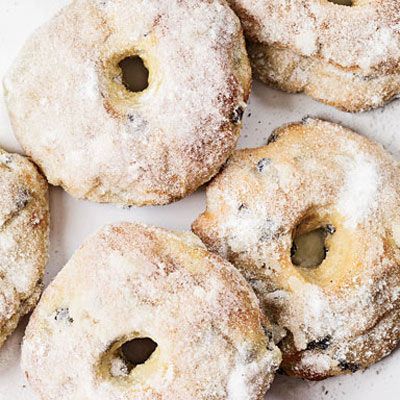The image features an overhead view of five doughnut-shaped pastries resting on a pale white surface, possibly a plate or table. These light-colored pastries, resembling doughnuts, are generously dusted with powdered sugar, making them appear slightly dry. Each pastry has a central hole, typical of doughnuts, but they are not perfectly round, adding a rustic charm. The pastries are speckled with small, dark berries which could be blueberries or chocolate chips. Crumbs are scattered around, enhancing the cozy, homemade feel of the image.